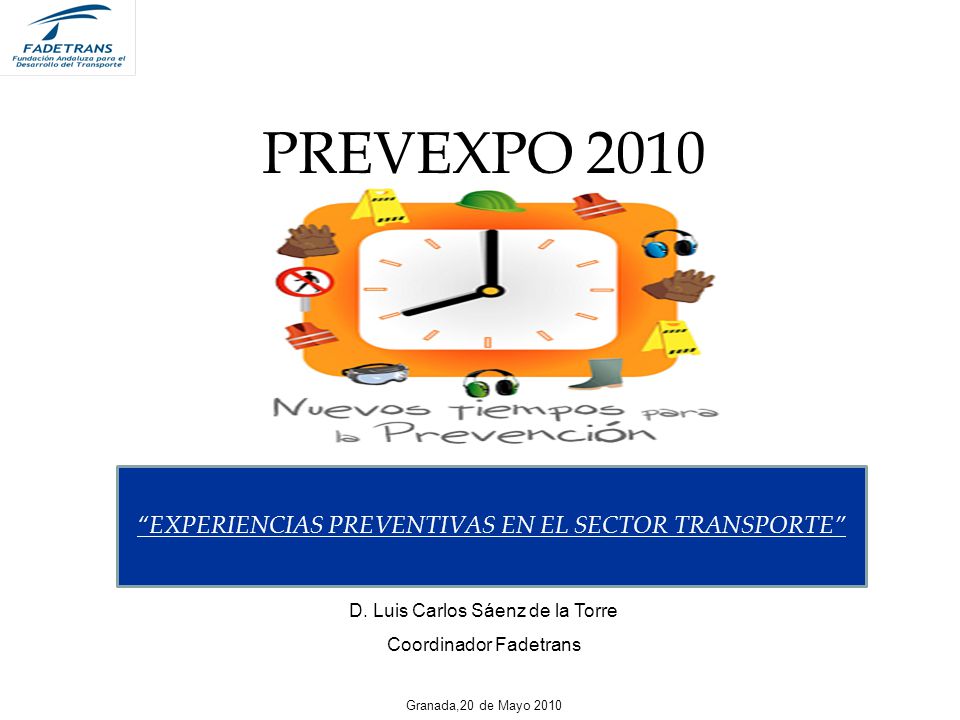The image is an advertisement, likely a slide from a slideshow, designed with a completely white background. In the upper left-hand corner, there is a white rectangle featuring a blue drawing of a tree and some text, one of which is "FADE TRANS," though the remaining text is too small to decipher clearly.

At the center, prominently displayed in bold black text, is the title "PREVEXPO 2010." Just below this, there is a cartoon-style drawing of an orange clock set to 7 o'clock. Surrounding the clock are various images of personal protective equipment (PPE), including a green hard hat at the top center, a red life jacket, blue headphones, brown gloves, a yellow caution sign, a work boot, additional pairs of headphones, safety glasses, another life jacket, a sign prohibiting walking with a red line through a person, and additional yellow caution signs.

Beneath this imagery, in black text, are the words "NUEVOS TIEMPOS PARA LA PREVENCIÓN," which translates to "New Times for Prevention." Below this phrase, a blue horizontal rectangle contains white text stating "EXPERIENCIAS PREVENTIVAS EN EL SECTOR TRANSPORTE," meaning "Preventive Experiences in the Transport Sector." Following this, in black text once more, the details "D. LUIS CARLOS SÁENZ DE LA TORRE, COORDINATOR, FADE TRANS," and "GRANADA, 20 DE MAYO 2010" are presented, indicating the presenter's name, title, and the date of the event.